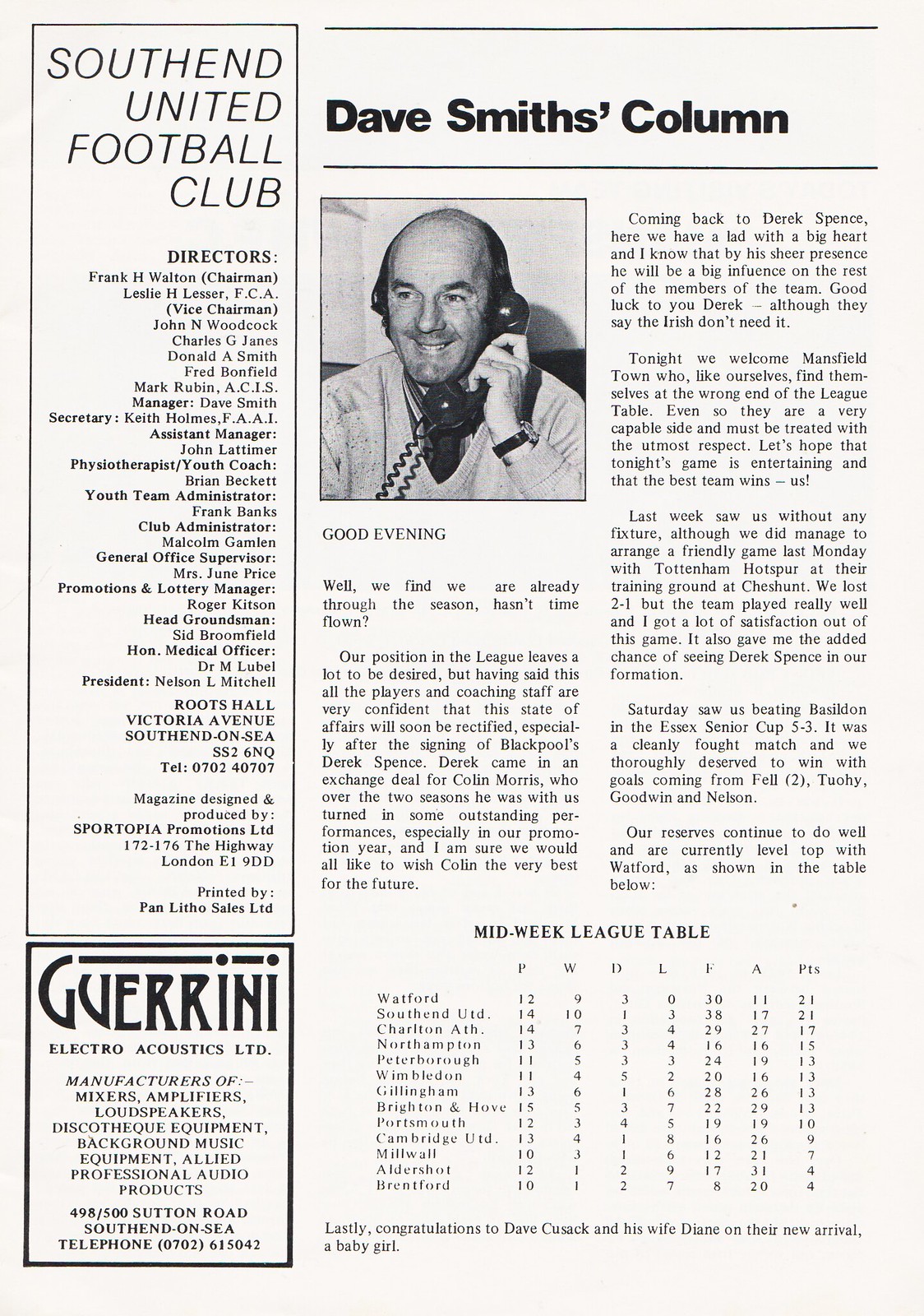The black-and-white image features a complex and detailed page from a sports newspaper or magazine. Dominating the right side is "Dave Smith's Column," illustrated with a photo of the bald gentleman holding a corded telephone and captioned "good evening." The column begins with a nostalgic reflection on the season's progress, noting "well, we find we are already through the season. Hasn't time flown?" Following the introductory remarks, the article extends into seven paragraphs and includes a midweek league table of games. At the conclusion of the column, a personal congratulatory note announces, "lastly, congratulations to Dave Cusack and his wife Diane on their new arrival, a baby girl."

Adjacent to the column, the left side of the page is dedicated to the South End United Football Club and lists numerous associated personnel, categorized into directors, managers, administrators, and groundsmen. The bottom of this section provides the club's address at Roots Hall, Victoria Avenue South, End on C, along with the telephone number 0702 40707. It's noted that the magazine is designed and produced by Sportopia Promotions Limited, with printing by Pan Litho Sales Limited.

Additionally, the bottom left corner displays a small advertisement for Guerini Electro Acoustics Limited. This ad promotes their range of professional audio products, including mixers, amplifiers, loudspeakers, and discotheque equipment, and lists their contact information at 498-500 Sutton Road, South End on C, Telephone 0702 615042.